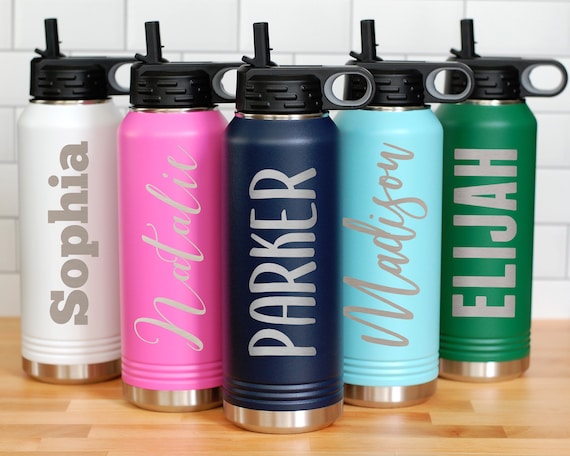This photo features five personalized water bottles, each with unique colors and names displayed on them, neatly arranged on a brown, butcher block tabletop. Behind the bottles is a backdrop of white subway tiles. All the bottles share a common design: a prominent silver bottom, black top with a sippy straw, and finger hold. From left to right:

1. A white bottle with the name "Sophia" written in white print.
2. A bright pink bottle with "Natalie" scripted elegantly in white.
3. A dark blue bottle in the center bearing the name "Parker" in white print.
4. A light blue bottle with "Madison" written in script.
5. A green bottle on the far right, displaying the name "Elijah" in white print.

Each bottle's name stands out in different fonts but consistently in a clean white color, making them easily distinguishable.